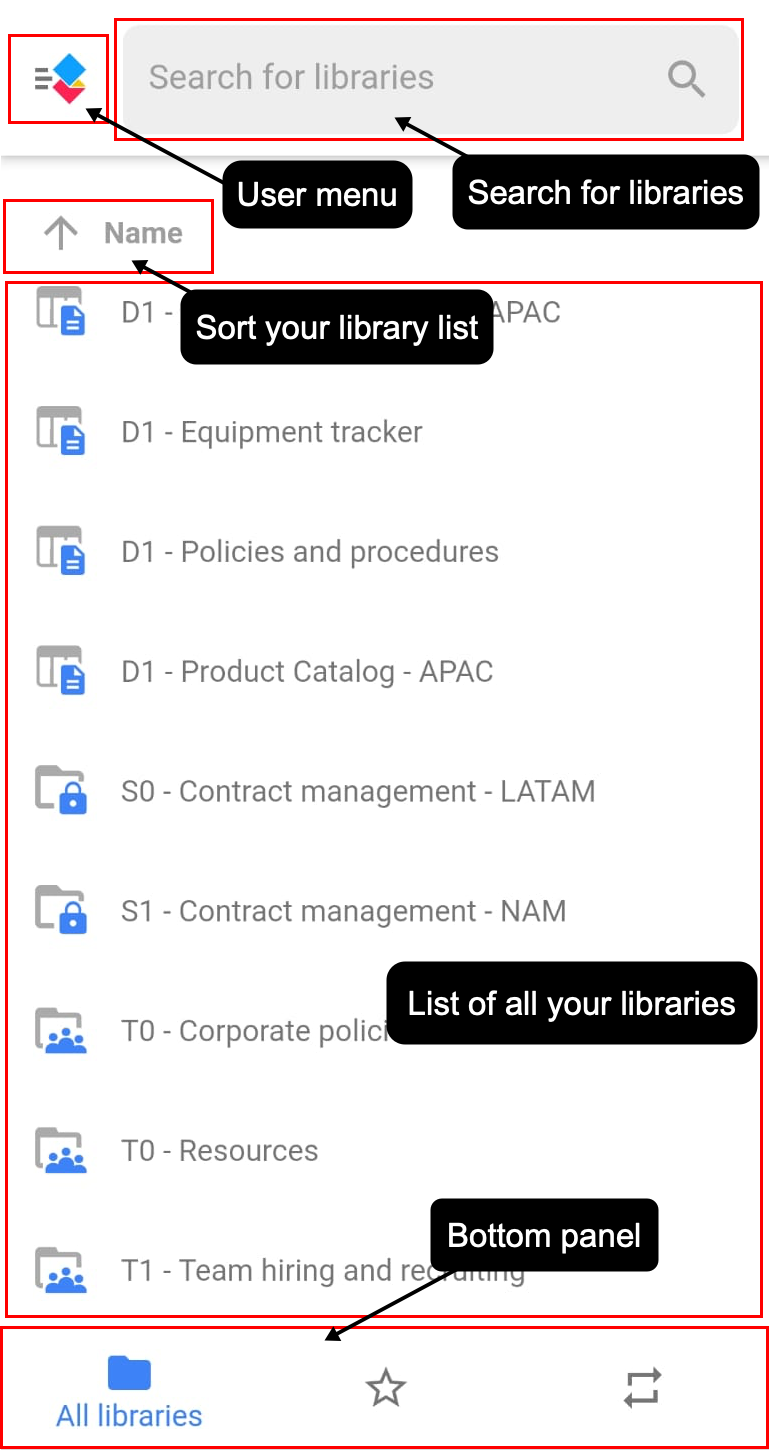A screenshot of a computer screen displaying a file sorting system or library management interface. At the top, there is a "burger" options icon, commonly used to represent a user menu, marked with a red outline and an arrow labeled "User Menu." Next to it, a search bar with the placeholder text "Search for libraries," also highlighted in red with an arrow labeled "Search for libraries."

Below the search bar is an upload icon (an upwards arrow) accompanied by the word "Name," highlighted with an arrow labeled "Sort your library list." Under this section is a list of files, each item outlined in red, and a black bar that reads "List of all your libraries." The files are as follows:
1. d1
2. d1 equipment tracker
3. d1 policies and procedures
4. d1 product catalog
5. a pack
6. s0 contract management
7. Lat am s1 contract management
8. am 2 contract policies
9. Resources
10. t1 team hiring and recruiting

At the bottom of the list is an "All libraries" option, a star icon, and a refresh button. The bottom panel of the interface is outlined in red with an arrow labeled "Bottom panel." The entire interface predominantly features gray or white text against a white background.